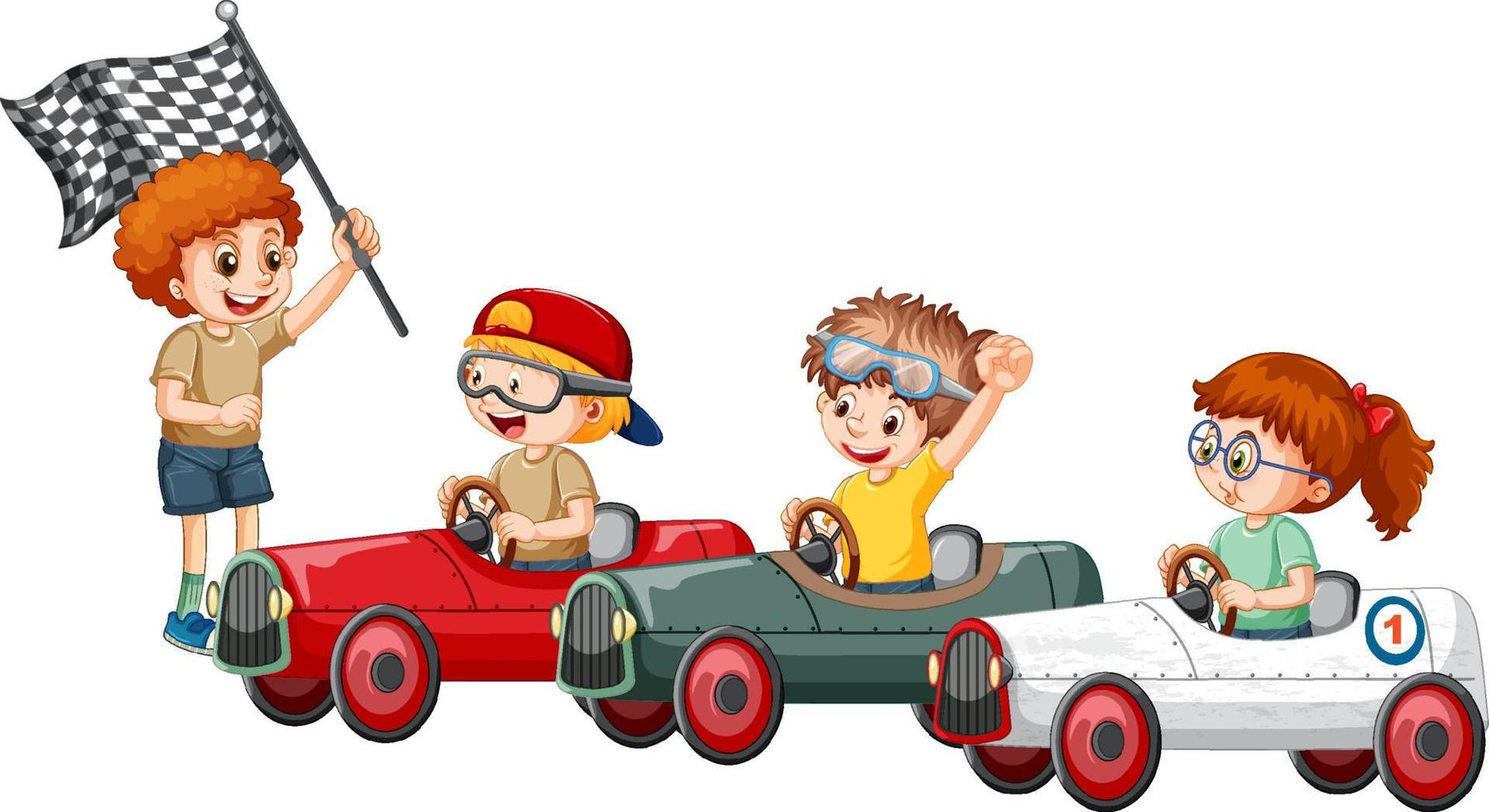This detailed cartoon features four children engaging in a whimsical go-kart race. On the far left stands a cheerful boy with curly red hair, holding a black and white checkered racing flag with a black flagpole. He is dressed in a tan t-shirt, blue shorts, green socks, and blue tennis shoes. This boy is depicted with a large smile and oversized eyes, adding to his animated appearance.

To his right sit three children in their respective go-karts, each uniquely detailed. The first child in a red go-kart sports a red baseball cap worn backward and protective goggles. He has short blonde hair and wears a beige t-shirt. This go-kart features red wheels, a gray seat back, and a grill with green accents, black and gray detailing, and two yellow headlights.

Next is a boy with brown, wavy hair and goggles perched above his eyes. He is clad in a yellow t-shirt and commands a green go-kart with red wheels, a gray seat back, and a matching grill design as the first, with black and gray colors and two yellow headlights.

On the far right, a girl with brown hair tied into a ponytail by a red ribbon drives a distinct white go-kart. She wears round glasses and a light green t-shirt. Her go-kart has red wheels and a grill surrounded by red accents, maintaining the black and gray grill design with two yellow headlights. A notable feature of her kart is a blue circle near the rear with a white center, emblazoned with the number one in orange.

Together, these elements create a lively and colorful representation of a children's go-kart race, filled with vibrant details and playful energy.